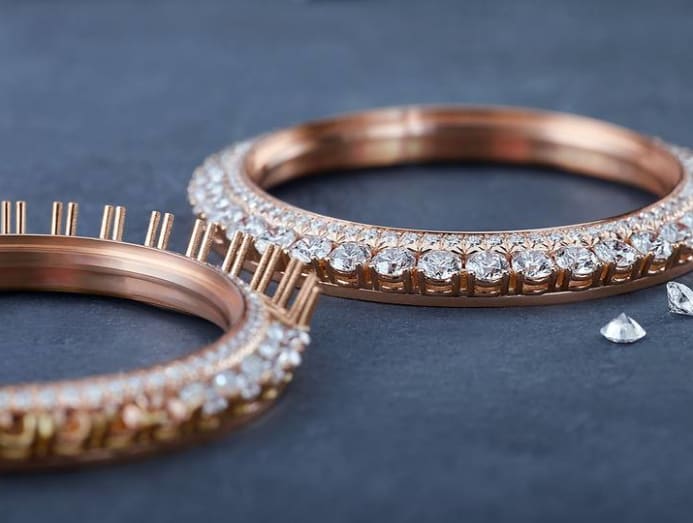This photograph showcases two rose gold diamond rings laid on a slate blue surface. The ring on the right side is a complete eternity band, featuring a pavé design with two rows of small round diamonds; one on the outer edge and another on the inside. Beside it, two loose diamonds suggest they might belong to this ring. The ring on the left is unfinished, with multiple prongs sticking up, waiting for diamonds to be set. While the photo is sharply focused in the middle, it blurs at the edges, adding an artistic touch to the detailed depiction of the jewelry.